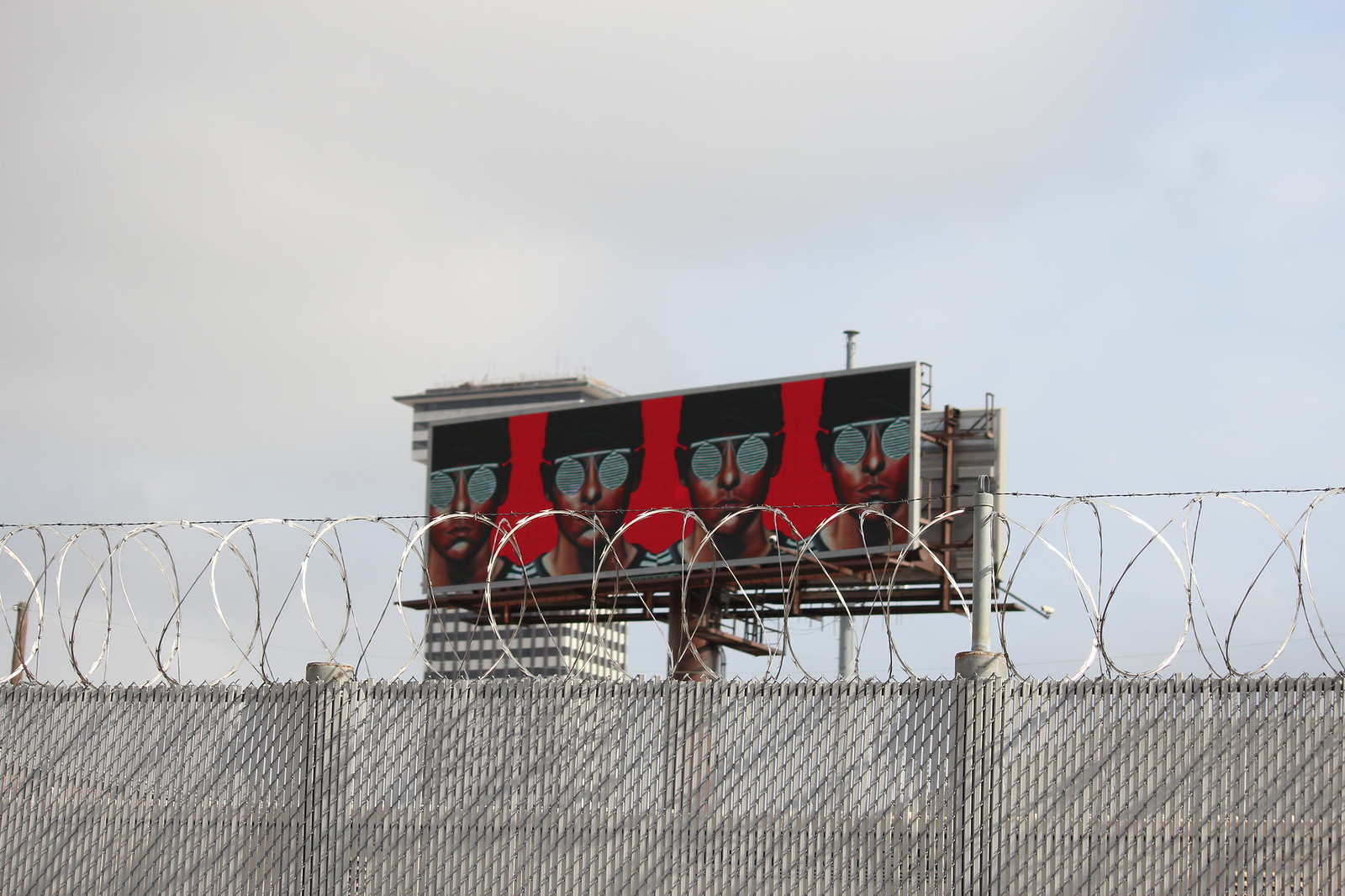In the foreground of the photo, a large chain-link fence topped with razor wire dominates the view, creating a sense of separation and security. Behind the fence stands a towering billboard positioned on a sturdy brown pole with a solid brown base. The billboard features a striking red background adorned with four identical faces of a person wearing round silver glasses, a black hat, and a striped shirt, repeated across the display. Looming behind the billboard is a structure resembling an airport control tower, adding an industrial feel to the scene. The sky above is mostly gray, with a hint of blue peeking through in the top right corner of the image. Just to the right of the main billboard, part of another billboard is visible, adding depth to the urban landscape.